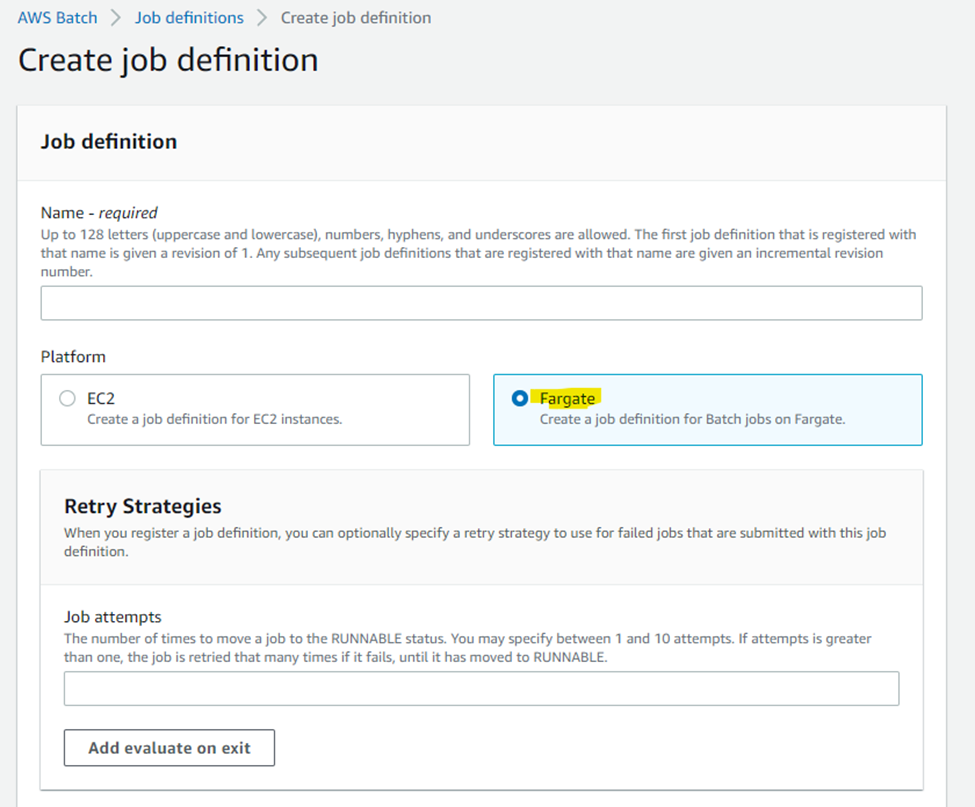Screenshot of the AWS Batch "Create Job Definition" Setup Page

At the top of the screenshot, the header reads "AWS Batch" in blue text, followed by a grey right arrow. To the right of the arrow is the text "Job definitions" also in blue, then another right arrow leading to "Create job definition." 

The main header below this is "Create job definition" in black. Beneath this header, there's an outlined area with a grey border on the right and left sides.

Inside this bordered area, the first section is labeled "Name (required)" with a description stating that the name can include up to 128 characters, combining uppercase and lowercase letters, numbers, hyphens, and underscores. It mentions that the first job definition registered with this name will be given a revision number of one, and subsequent job definitions will receive incremental revision numbers. Below this description, there is a large input field for entering the name.

Further down, there are two radio button options under the "Platform" section. The left option reads "EC2" with a description to create a job definition for EC2 instances. The right option shows "Fargate" and is highlighted in yellow, indicating it is selected. This option is for creating job definitions for batch jobs on Fargate. The selected area is also denoted by a blue outline.

Below the platform section, there is a segment titled "Retry strategies." It explains that when registering a job definition, you can specify a retry strategy to be used if jobs fail. Another sub-section under this is "Job attempts," detailing that the number of attempts can be set between one and ten. If set to more than one, the job will be retried the specified number of times if it initially fails and moves to the runnable status. There is an empty field for specifying job attempts below this description.

At the bottom left of the screen is a button labeled "Add evaluate on exit."

This screenshot provides a detailed overview of the steps and options available while creating a job definition in AWS Batch, showing features such as naming conventions, platform choices, retry strategies, and job attempt configurations.